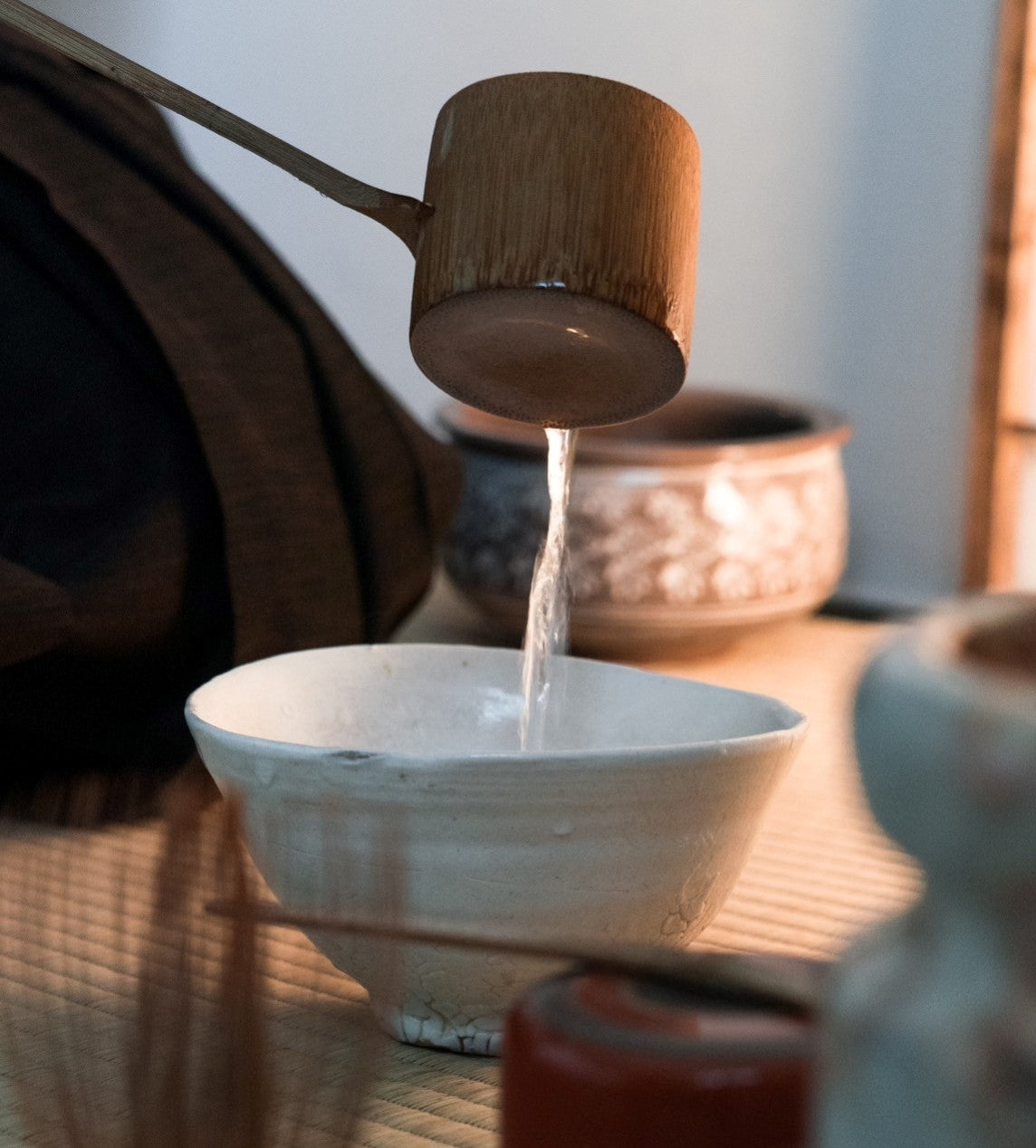This close-up portrait image features an artful arrangement of ceramic ware set against light blue walls. Center stage is a small, handmade white ceramic bowl with subtle brown stripes. A finely crafted wooden ladle is gracefully pouring water into this bowl. 

In the background, a larger, brown ceramic bowl adorned with white decorations is partially visible. The foreground reveals a blurred taller vase and a smaller red ceramic piece topped with a wooden tool, possibly indicative of traditional craftsmanship. 

Adding to the composition, straw-like elements—perhaps a plant or a brush—are seen emerging. The scene is set on a striped reed or bamboo mat, enhancing the earthy, artisanal vibe. An additional dark brown fabric, possibly a bag, is discernible in the background, adding depth to this serene depiction of ceramic artistry. Peeking from the scene’s edge, a window frame further contextualizes the space.